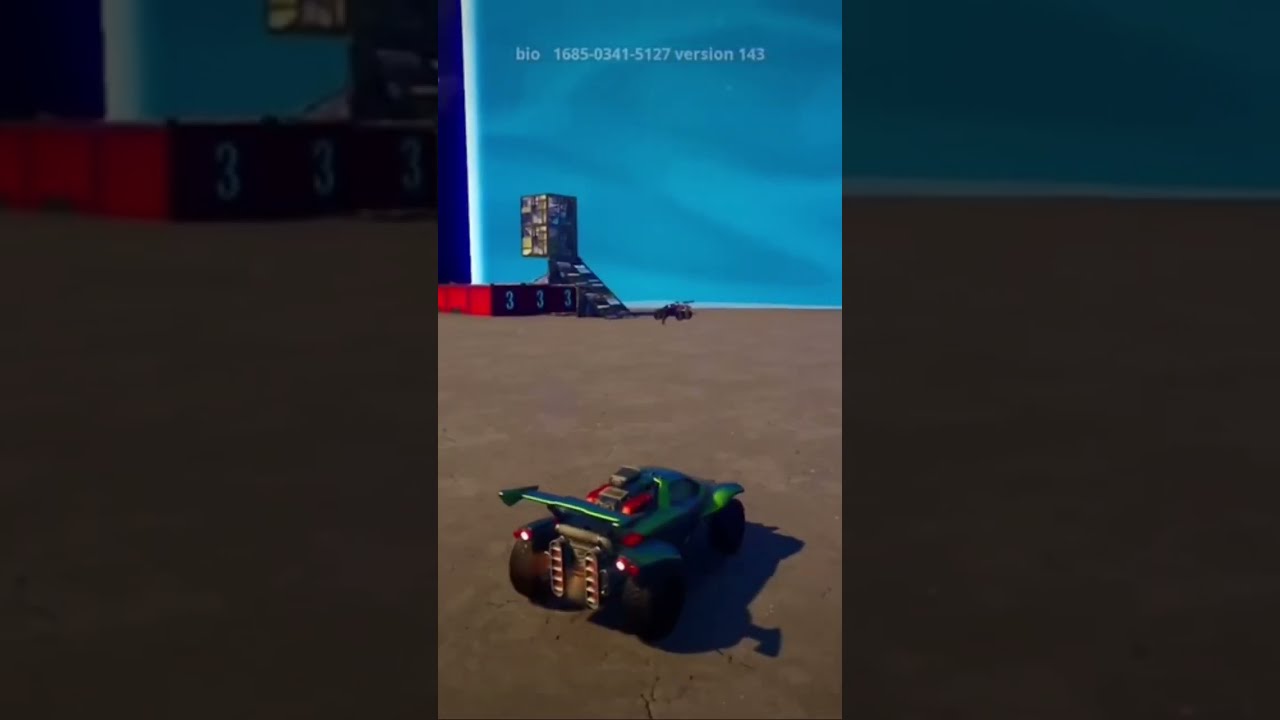The image depicts a scene that seems to be a screen grab from a video game, characterized by its distinct, almost convincing 3D elements. Dominating the foreground is a small green sports car with red accents, resembling a remote-controlled (RC) car. It casts a dark black shadow on a brown, cracked concrete surface, further enhancing its realism. The car’s backlights are turned on, adding to the detailing.

In the background, the scene transitions into a more artificial and less convincing setup. There’s another RC-like vehicle, positioned on a structure composed of block-like platforms. Notably, one platform to the left is a red-bottomed muscle box marked with white "333" numbers, and another to the right appears serrated, hinting at a racing environment. The backdrop features a sky image, giving it a staged look, and includes a teal-colored square at the top displaying the text “BIO 168503415127 version 143.” The overall setting appears to be a rocky, desert-like field, with a mixture of grays, blues, and browns defining the different surfaces and structures, contributing to the video game's simulated racing atmosphere.